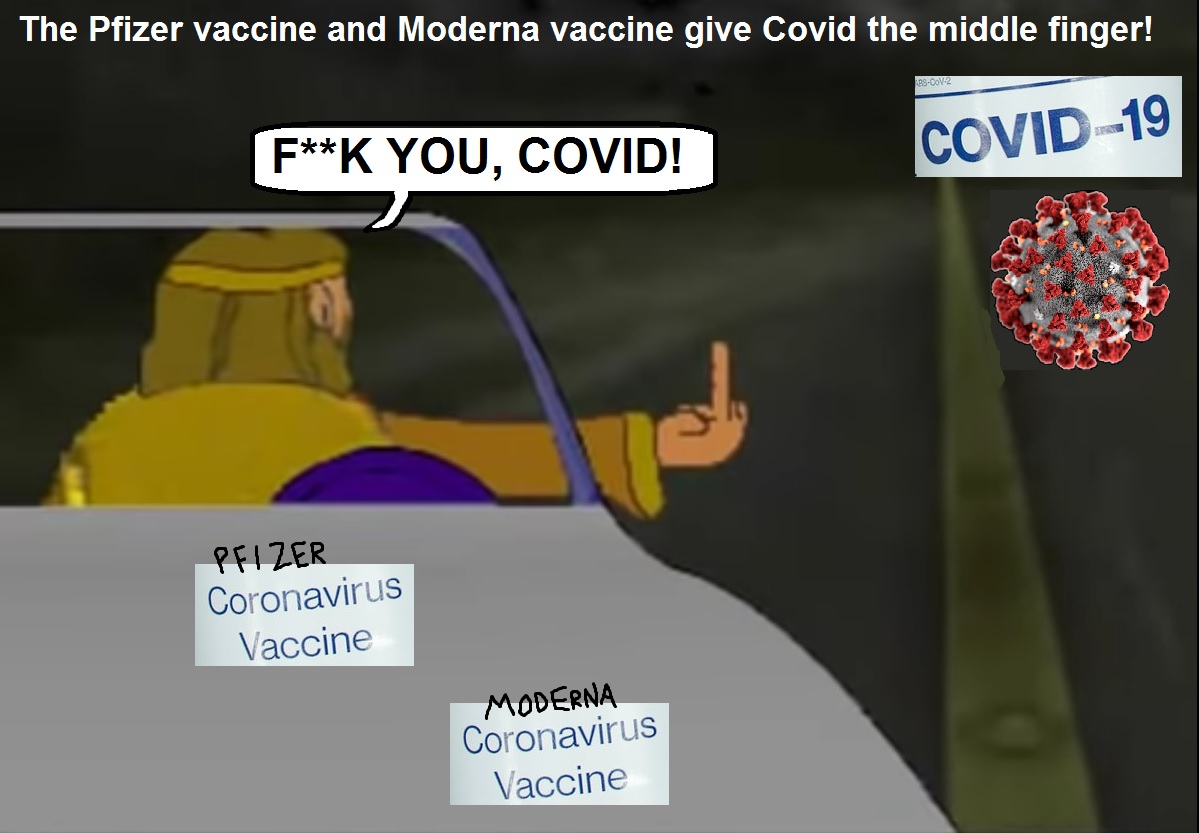The image is a heavily edited meme illustration featuring a cartoon depiction of a car on the left side. Inside the car, a person wearing yellow robes with long sleeves and a yellow headband is seated in the driver’s seat. The person has their right hand out of the window with their thumb and three fingers curled in, except for their middle finger which is pointed straight up. Above the scene, white text reads, "The Pfizer vaccine and Moderna vaccine give COVID the middle finger." A speech bubble from the person in the car says, "F**K U COVID!" On the car’s hood, there is a white rectangle labeled "coronavirus vaccine" in blue with "P-F-I-Z-E-R" handwritten above it. To the right side of the image, there is a white sign that says "COVID-19" next to an illustration representing the COVID-19 virus molecules. The overall layout has the car covering the lower left quadrant, making it the central focus along with the defiant gesture directed toward COVID-19.